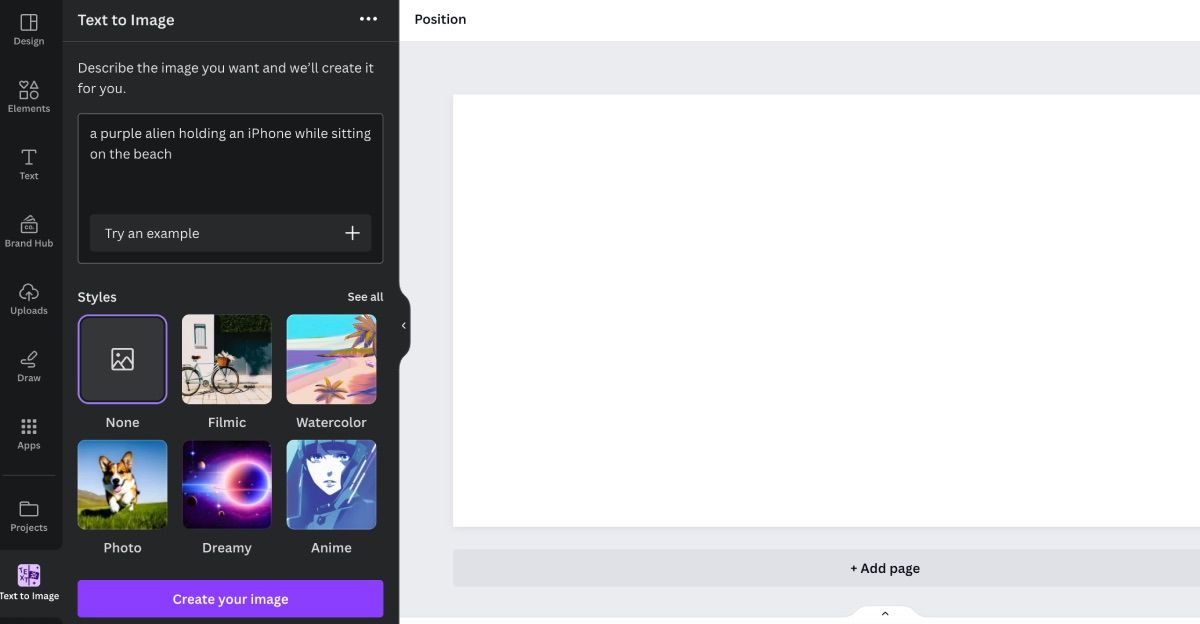This image showcases a user interface for a text-to-image generation tool. The left side of the image features a dark background, almost black, extending from the top to slightly past the center. A vertical menu is positioned on the left-hand side, presenting a sequence of options from top to bottom: "Designs," "Elements," "Text," "Brand Hub," "Uploads," "Draw," "Apps," and "Objects." Immediately to the right of the menu, the interface prominently displays a white square area labeled "Text to Image." Above this section is an instructional prompt: "Describe the image you want and we'll create it for you." Below the prompt is an input text box where users can type their image descriptions. The overall layout employs a clean and intuitive design, organized to facilitate an efficient user experience in generating images from textual descriptions.